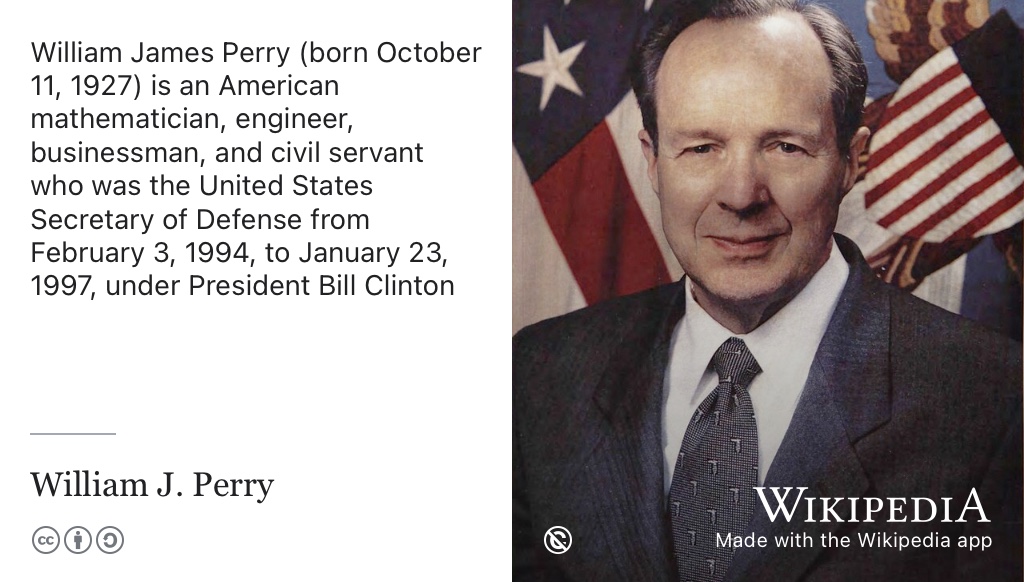The image shows a Wikipedia article as displayed in the Wikipedia app, featuring a close-up portrait of William James Perry, a prominent American figure. The article's text is on the left side, set against a white background with black print. On the right side of the app, it indicates the content is from Wikipedia, made using the Wikipedia app. The portrait captures Perry from mid-chest up; he has short brown hair and is looking directly at the camera. He is dressed in a gray suit jacket, a white collared shirt, and a greenish tie. The background includes red, white, and blue elements of the American flag, symbolizing his political role. The caption next to his portrait reads: "William James Perry, born October 11, 1927, is an American mathematician, engineer, businessman, and civil servant who was the United States Secretary of Defense from February 3, 1994, to January 23, 1997, under President Bill Clinton." At the bottom of the caption, it simply states "William J. Perry," and there are various circular icons, possibly for sharing the content.